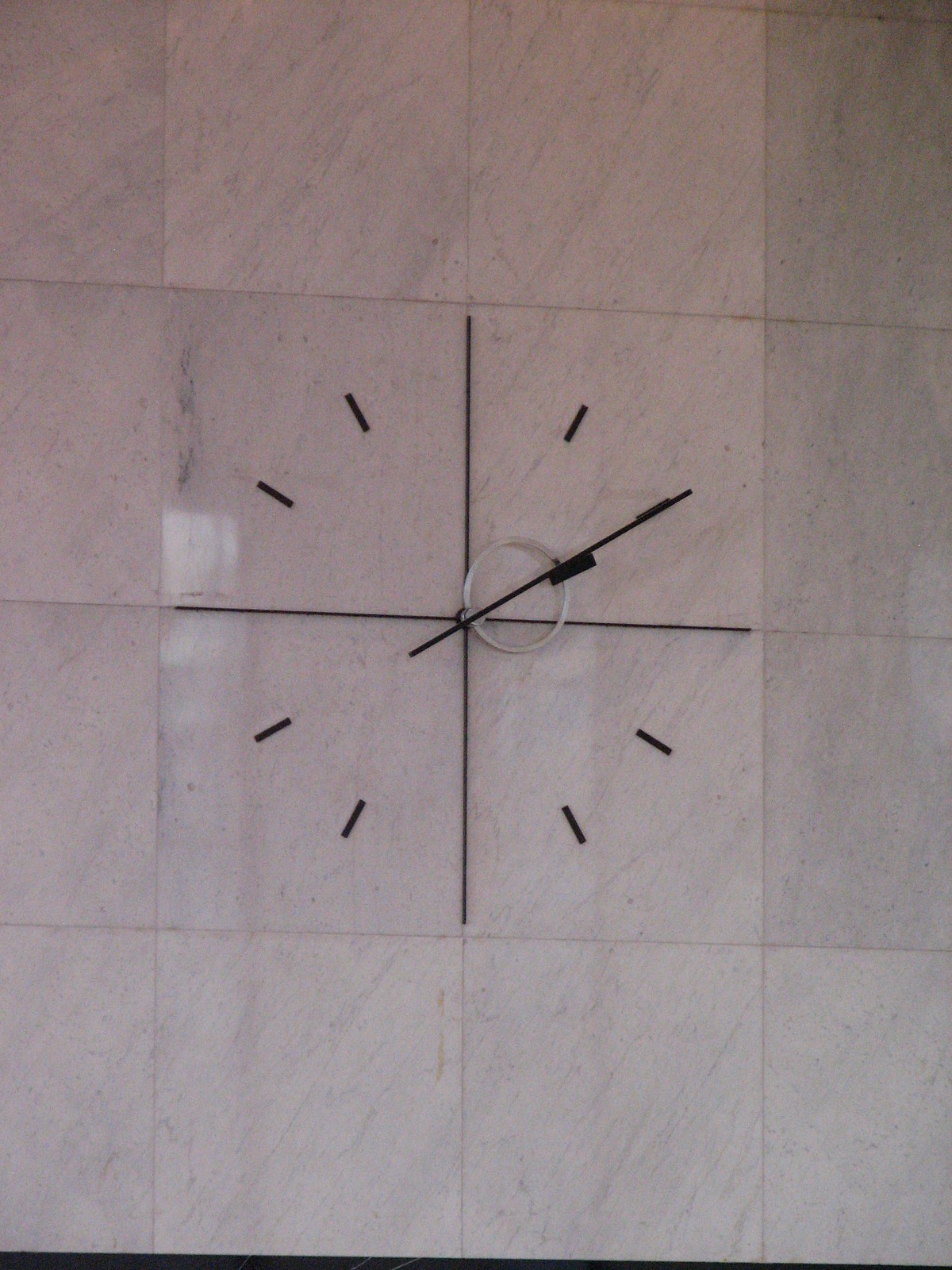This indoor photograph showcases a section of a marble wall adorned with a simple yet elegant clock. The wall is composed of square tiles arranged in a grid, with four rows and four columns visible. The tiles extend beyond the photo's edges, creating an uninterrupted marble pattern. Dominating the photo's center are four marbled gray and white tiles, distinguished by their veined texture.

Mounted directly on these tiles is a minimalist clock. Its face, marked by clean, straightforward design, features lines denoting the numbers in a circular arrangement. A sleek black minute hand and a black hour hand with a gray circular base grace the clock, complementing its subdued aesthetic. Moreover, two thin black lines form a cross, extending horizontally from the 3 to 9 positions and vertically from 12 to 6, adding a touch of geometric precision to the overall composition.